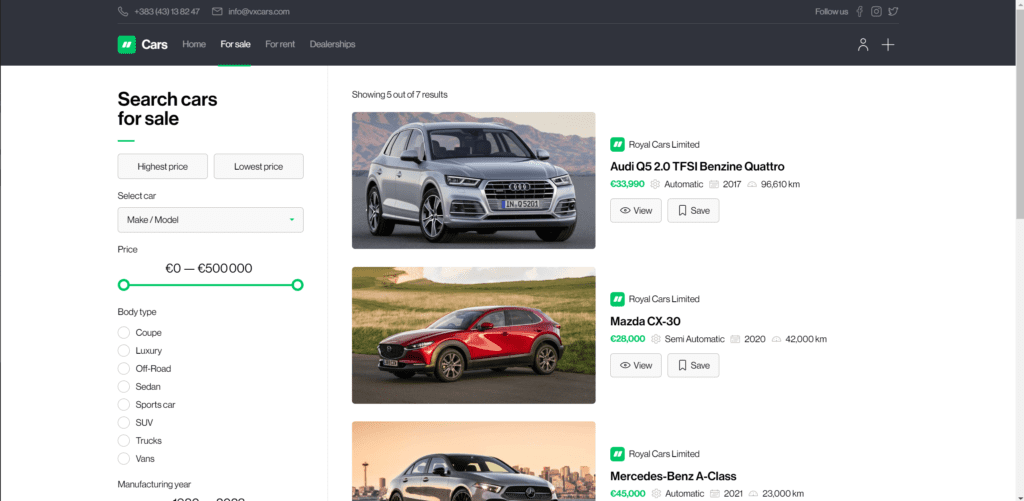The webpage from CARS.com features a sleek design with a prominent black banner at the top. Positioned on the upper left is a phone icon accompanied by contact details, including a phone number and an email, info@CARS.com. On the far right, social media icons for Facebook, Instagram, and X invite users to connect. Below, a user icon with a plus sign indicates membership or account options.

The main navigation bar includes a bold white "CARS" logo set beside a green box containing white quotation marks. To the right are links for "Home," "For Sale," "For Rent," and "Dealerships," with "For Sale" currently selected.

The page itself has a clean white background with a central column showcasing three vehicles for sale, each represented by an image. The sidebar on the left begins with a "Search Cars for Sale" header in black, featuring input boxes for highest and lowest price filters. There is also a dropdown menu for selecting car make and model, a sliding bar for price range, and a vertical list of body type options in gray text, including Coupe, Luxury, Off-Road, Sedan, Sports Car, SUV, Trucks, and Vans. Additionally, users can specify the manufacturing year.

The highlighted vehicles in the listings are an Audi Q5 2.0 TFSI Benzine Quattro, a Mazda CX-30, and a Mercedes-Benz A-Class.